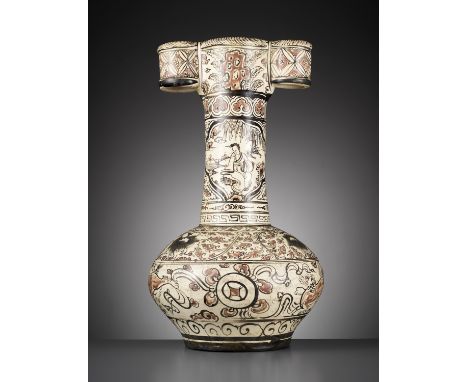This photograph captures an ornate, ancient vase set against an abstract gray background with a gradient effect, darker at the edges. The vase, which sits on a gray table, appears to be illuminated by a spotlight that highlights its intricate features. The main body of the vase is a tan or beige color adorned with black and red floral prints and geometric shapes. Central to the vase's design is an image of a man meditating in water, surrounded by Chinese symbols, suggestive of Chinese art. The vase has a bulbous bottom and a tall, tubular top with two cylindrical handles extending from the sides. The vase's reflective surface adds to its visual appeal, making it a striking subject against the contrasting background.